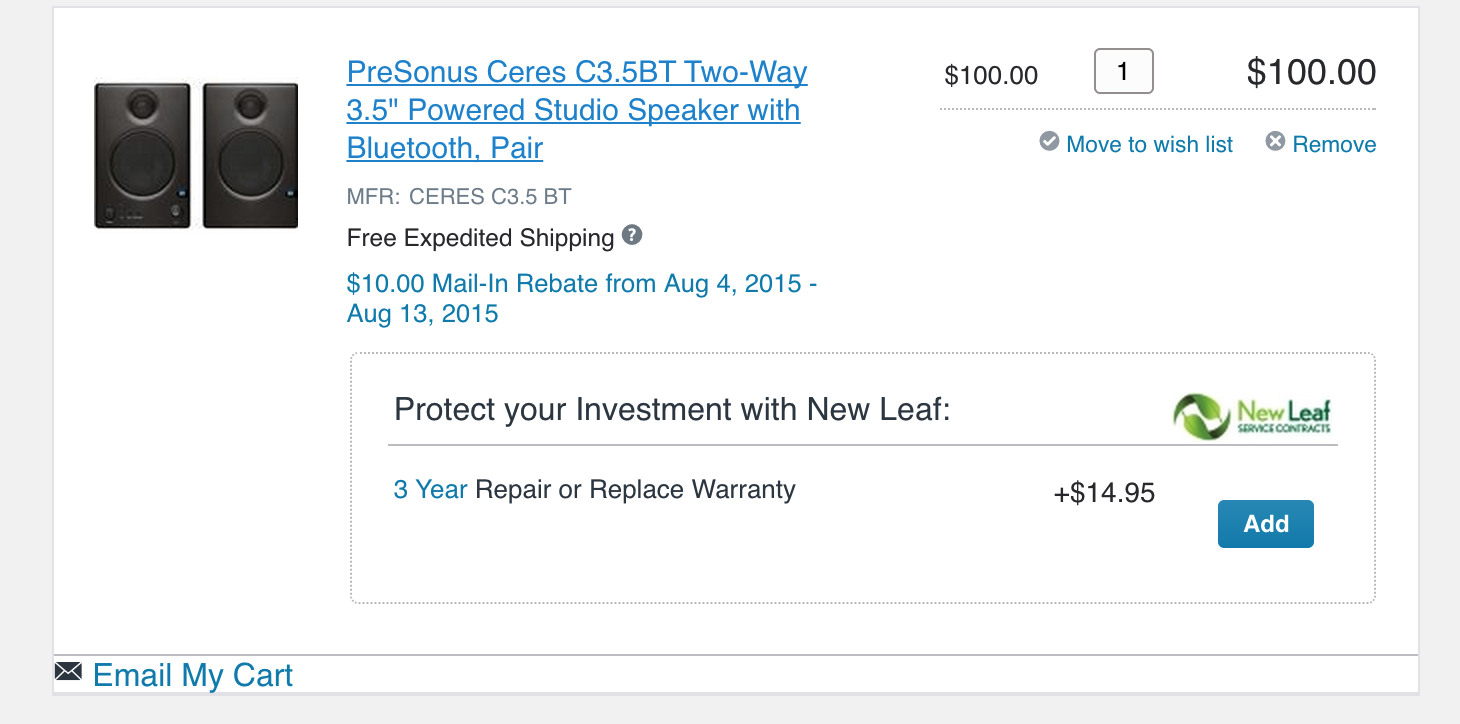In this screenshot of an online shopping cart, we see a white-background interface displaying two speakers prominently on the upper left. To the right of the speakers, the product description is rendered in blue underlined text, reading "Three Sonos Ceres C3.5BT two-way 3.5 inches powered studio speaker with Bluetooth pair." Directly below this in gray text is "MFR: Ceres C3.5BT," followed by "free expedited shipping" written in black. Additionally, there is a promotional offer in blue text, stating, "$10 mail-in rebate from August 4, 2015 to August 13, 2015." On the lower right side of the screenshot, there is a conspicuous blue "Add" button with white text.